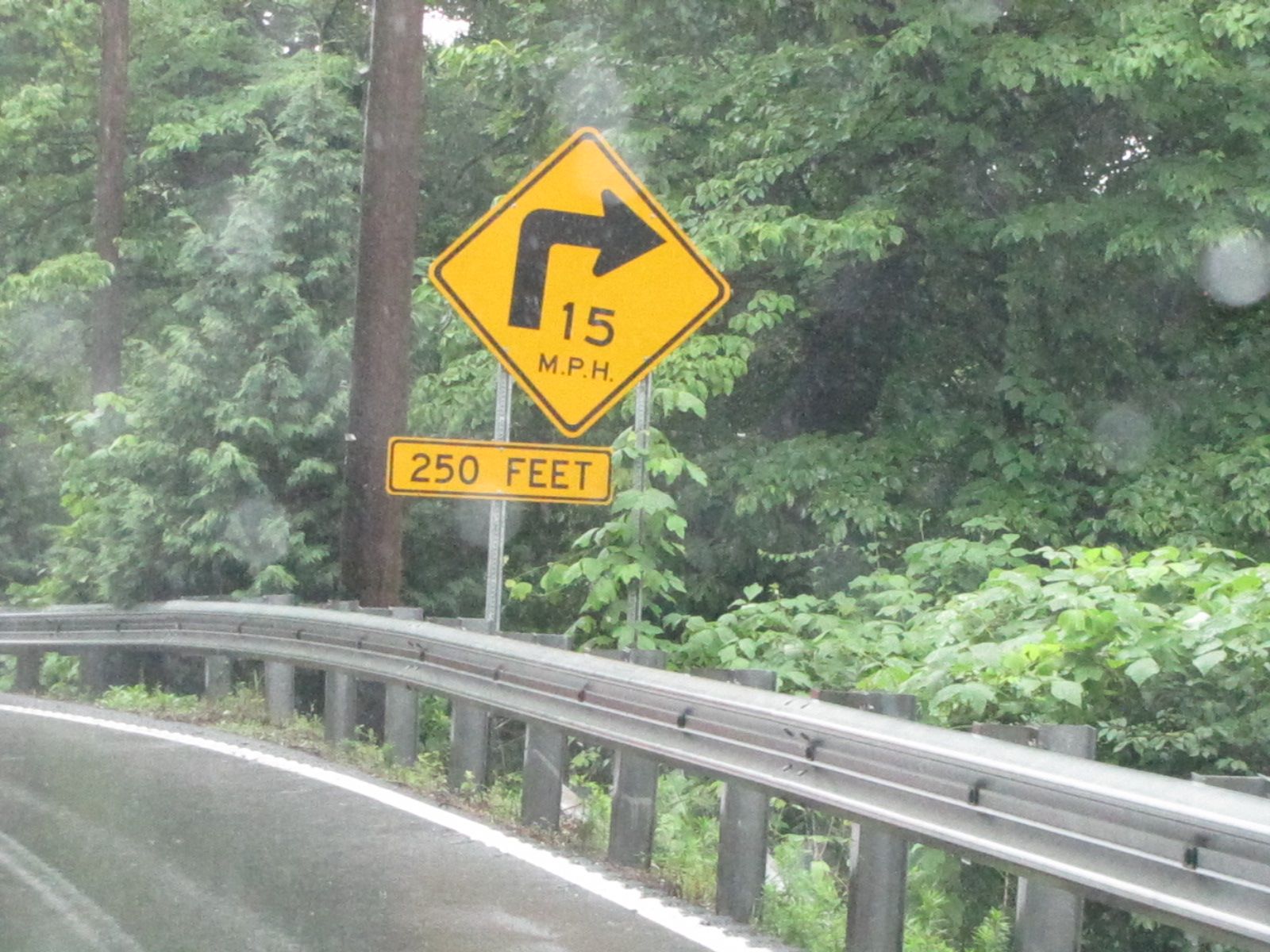This photograph captures a road sign situated in a wooded area. Dominating the center is a yellow diamond-shaped sign with a black border, featuring a bold black arrow that curves to the right. Beneath the arrow, "15 M-P-H" is clearly printed in black. Directly underneath this sign, a smaller rectangular yellow sign reads "250 feet," also in black. Both signs are supported by two steel posts.

To the left of the signs, there's a brown telephone pole, with another visible further down the left side. A silver guardrail, held up by vertical metal supports bolted at regular intervals, stretches diagonally across the lower portion of the image from the lower right to the lower left. Adjacent to the guardrail on the left is a white line marking the edge of a gray asphalt pavement.

The background consists of a dense array of trees and green foliage, adding a lush natural backdrop to the scene.